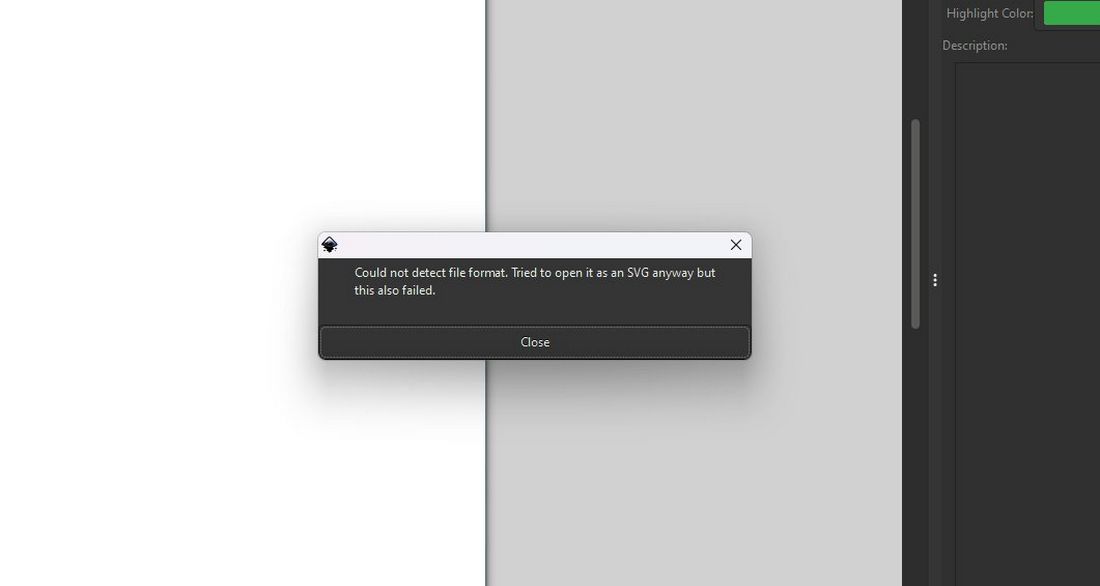The image primarily features a pop-up error message at its center, surrounded by an indistinct background hinting at a software interface or website. The pop-up message is the focal point, characterized by a white bar at the top. In the top left corner of this bar, there is an odd-looking diamond symbol, while the right corner houses a standard 'X' for closing the pop-up. 

Below the bar, the message area starts with a dark gray to black background, displaying a concise error message in small white letters: "Could not detect file format. Tried to open it as an SVG anyway but this also failed." 

At the bottom of the pop-up, a 'close' button spans the entire width. The pop-up itself is accentuated with a large, blurry drop shadow. 

The immediate backdrop isn't clearly identifiable but features a noticeable change in color. To the left of the pop-up, there is a white background, while the right side reveals a strip of a gray background with another drop shadow. Beyond this, to the far right, you can make out the left edge of the encompassing interface, predominantly black. At the top left of this area, the text "Highlight Color" and a green icon are visible. Below that, the word "Description" appears above a large text field. The rest of the image’s details are vague and indiscernible.